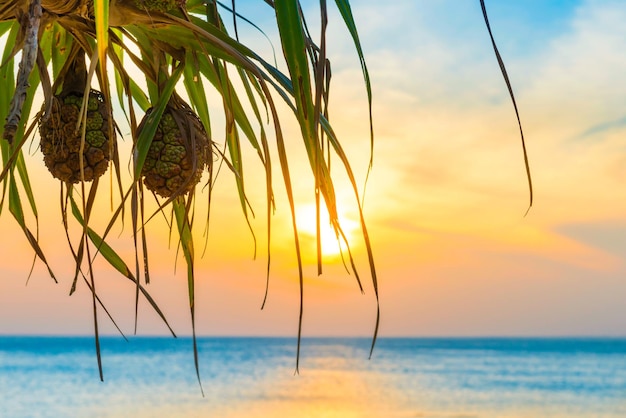The photograph captures a vibrant tropical beach scene with a clear blue sea at the bottom and a bright, sunny sky. Dominating the foreground on the left are two large, brown, oval-shaped coconut-like fruits hanging from a branch with green, slender palm fronds. The sun, positioned centrally behind the leaves, is bright yellow, casting a radiant light that diffuses into pinkish, orange, and blue hues across the sky and horizon. White, fluffy clouds hover in the blue expanse above. The overall setting conveys a refreshing, tropical paradise with rich colors and serene natural elements.